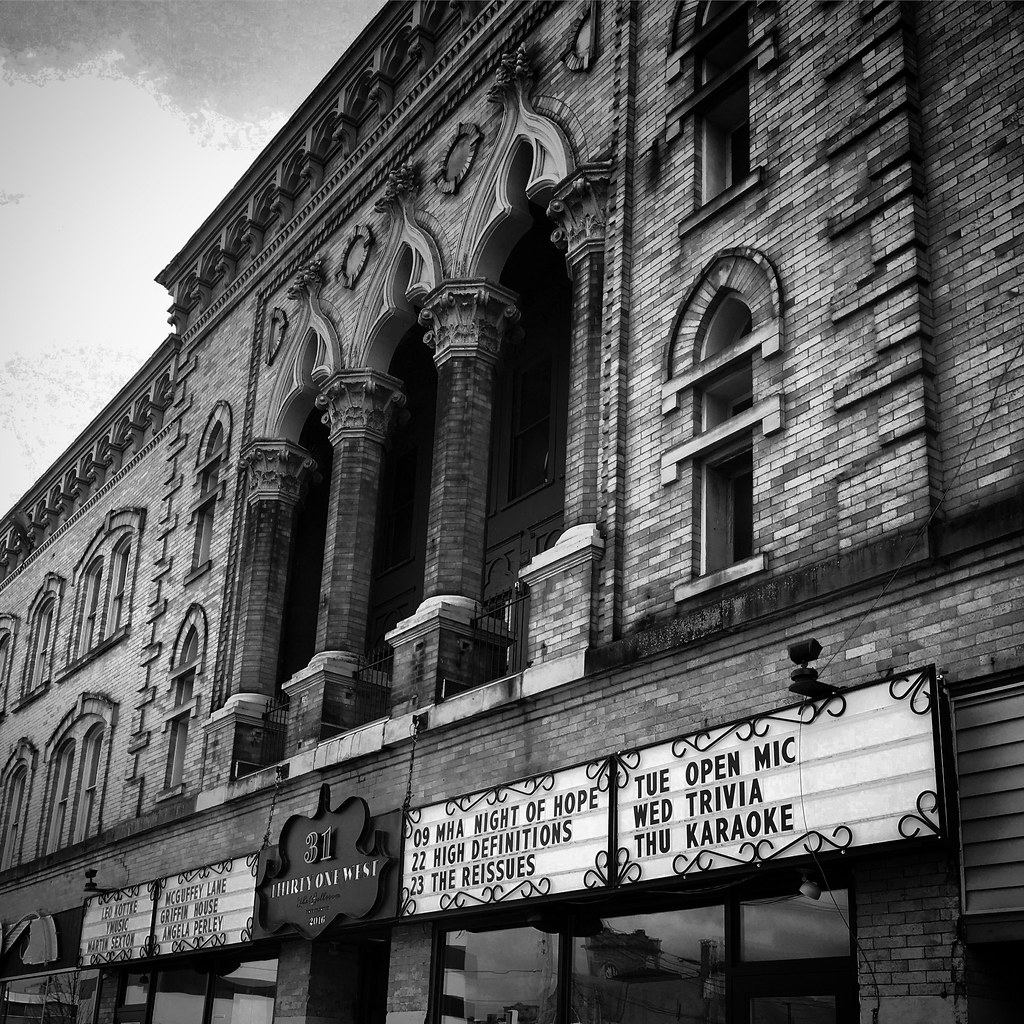This black-and-white digital photograph captures an imposing and very large, three-story theater building made entirely of brick. The image is taken from a low angle at approximately a 45-degree perspective from the right side, emphasizing the building's height and grandeur. The intricate Victorian architectural elements are evident, with prominent stone columns and ornamental designs near the top. The theater features a series of modern windows on the lower levels and older arch-topped windows higher up.

Centered at the building's front is a black, flower-shaped sign bearing the number '31' with some illegible text beneath it. Flanking this central sign are four marquee-style signs, two on each side, resembling classic cinema or theater signs where letters can be slid in to display messages. The legible text on these signs includes phrases such as "Night of Hope," "High Definitions," "Tuesday Open Mic," "Wednesday Trivia," and "Thursday Karaoke." Additionally, there's a placard near the base of the building that reads '41 West.' This combination of historic architecture and modern signage creates a striking visual contrast, emphasizing the theater's longstanding presence and current cultural offerings.